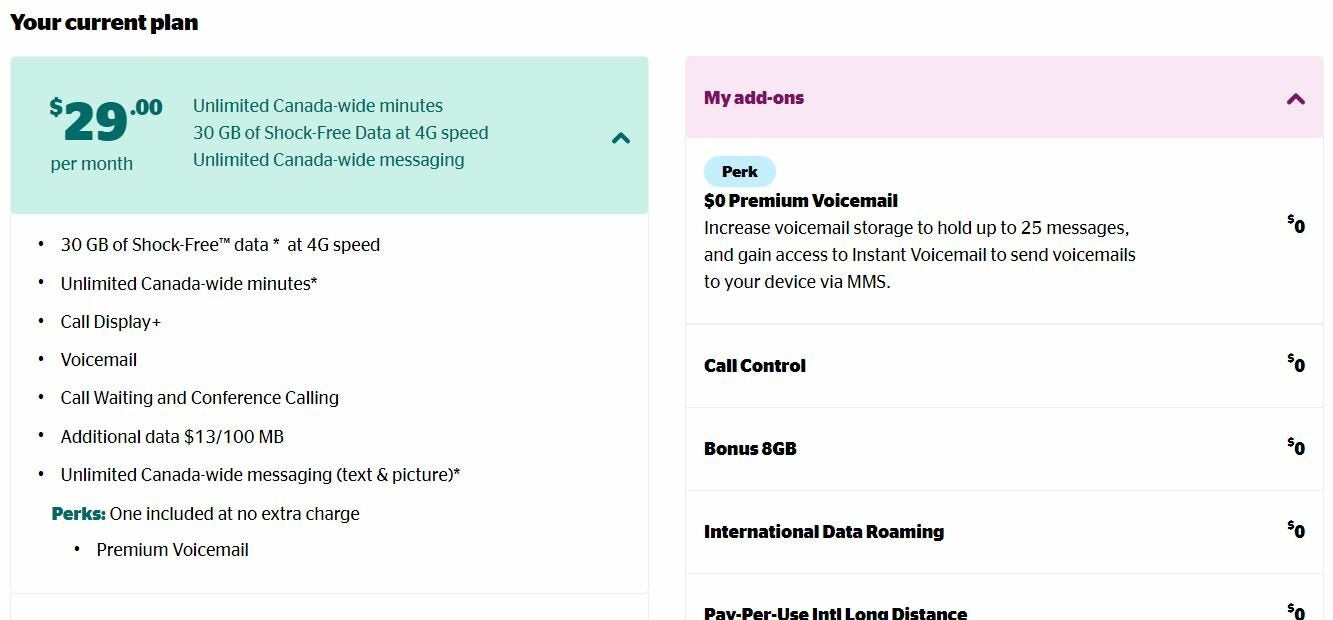The image is a screenshot of a web page used for selecting a wireless connectivity plan. The background of the page is white, and it is divided into two distinct sections. The left side of the page features a headline in black font that reads "Your Current Plan." Below this headline, there is a light aquamarine green rectangle that holds the key details of the plan in a slightly darker aquamarine font. Highlighted prominently in bold is "$29 per month," and beside it, the plan offers "Unlimited Canada-wide minutes, 30 GB of shock-free data at 4G speed, and Unlimited Canada-wide messaging."

Directly underneath this aquamarine section, on a white background with dark gray font, additional plan details are listed. These include features mentioned before, as well as new items such as voicemail, call waiting, and conference calling. It specifies that voicemail data costs $13 per 100 MB and reiterates Unlimited Canada-wide messaging for text and picture. The word "PERKS" appears in the same aquamarine font with a note stating "one included at no extra charge." The list concludes with "premium voicemail."

On the right side of the page, a separate column begins with a very light lavender rectangle at the top. Written in purple, it says "My Add-Ons." The first add-on listed is "$0 premium voicemail," which includes increased voicemail storage for up to 25 messages and instant voicemail access via MMS. This column continues with other add-ons, all listed in bold black font and showing a $0 cost on the right side. These add-ons include "call control," "bonus 8 GB," "international data roaming," and "pay-per-use international long distance."